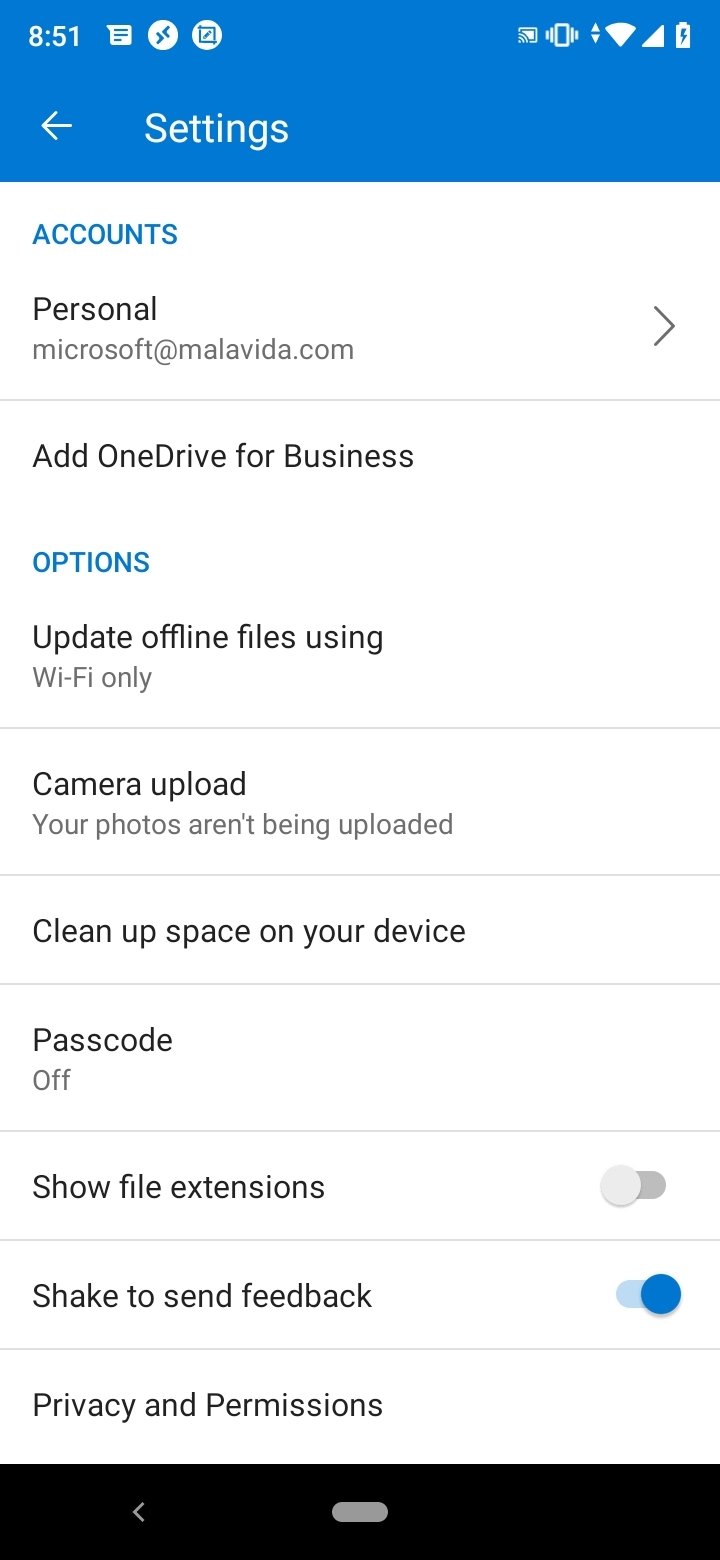The image depicts the settings screen of an application on an Android smartphone, characterized by its distinct blue top banner and white iconography against the blue background. The phone's heads-up display shows full Wi-Fi and cellular service, a full battery, and silent mode enabled. Several app notifications, including messages, are visible on the left side of the status bar.

The settings screen itself is presented on a white background with a structured layout. At the top, the section labelled "Accounts" appears in blue text, indicating the user's personal email account beneath in black text. An arrow to the right suggests additional options are accessible.

Below this, separated by a divider, are the following options: "Add to OneDrive for Business" with clickable blue text, "Update Offline Files," "Camera Upload," "Clean Up Space on Your Device," and "Passcode Off." Each option is clearly demarcated by dividers.

Further down, two toggles are available - "Show File Extensions" (currently off, displayed in gray) and "Shake to Send Feedback" (currently on, displayed in blue).

At the bottom, the section "Privacy and Permissions" is present, presumably a clickable option, completing the settings screen. The screen ends with a black banner housing the Android navigation buttons.